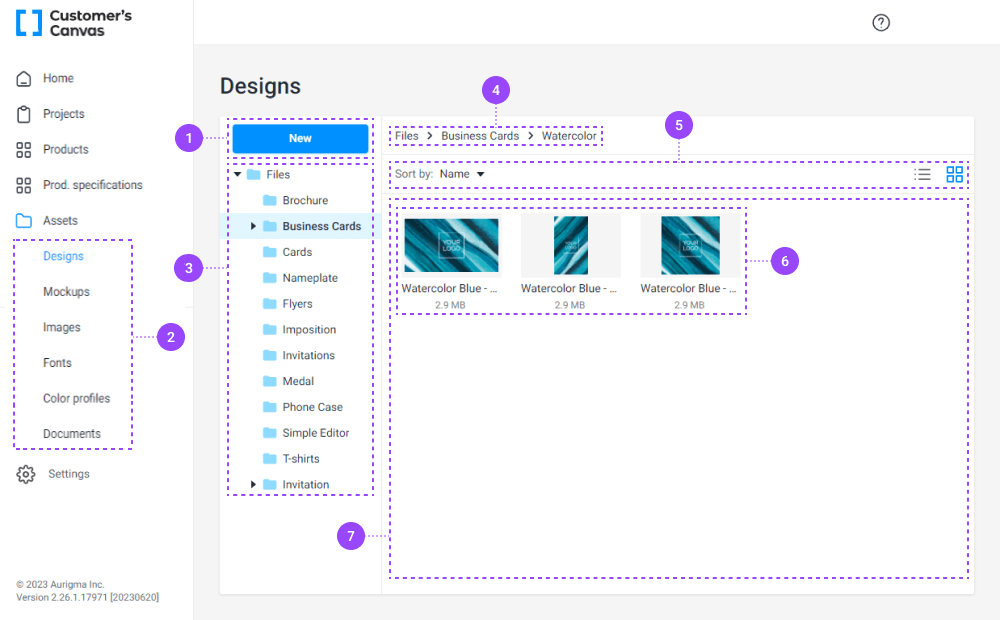The image features a layout divided into two sections, distinctly separated by a thin green line. On the left side:

- The background is primarily white, with the top left corner featuring a broken outline of a blue rectangle, creating an impression of fragmented contour lines.
- Adjacent to this, in black text, it reads, "Customer's Canvas." Below this, another black text signifies "House for a Home."
- A dotted purple line rectangular box within this area contains various labels. In gray, it lists "assets," while in blue, it mentions "designs." Additional gray labels include "fonts," "images," "color profiles," and "mock-ups."
- Extending from the right side of this rectangle, there is a dotted line connected to a purple circle. Inside the circle, it reads "to" in white text.
- Further to the right, the gray text continues to list items: "projects," "products," "specifications," "editors," "PM," "products," "payment," and "workflow settings."
- At the bottom of this section, it notes "2003 Arigma Inc." and a version number "2.26.1.17971."

On the right side of the layout:

- The black text at the top announces "designs." This section also features a series of dotted rectangles organized in a list format.
- The first rectangle has the number "one" linked with a "three," accompanied by a blue "new" label.
- Following this, in black text, are labels for "files," "brochures," "business cards" (with "cards" highlighted in blue), "nameplate," "flyers," "position," "invitation," "medal," "phone case," "simple," "editor," and "t-shirt invitation."
- Another dotted purple box, marked with the number "four," also lists "files," "business cards," and "watercolor."
- Yet another rectangle, numbered "five," is labeled "short by name."
- Finally, the last set of boxes features a dual-layer structure: an outer dotted box labeled "seven" with an inner box labeled "six."

This detailed and structured layout visually organizes the subjects and categories of the interface.